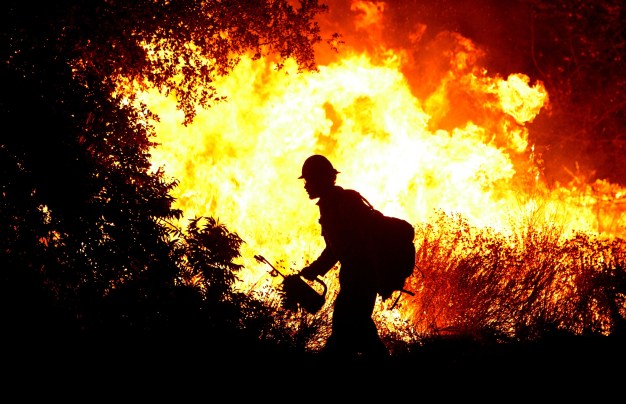A dramatic nighttime scene captures a man in silhouette, standing amidst a fierce blaze. The fire, with intense, towering flames in bright yellow, orange, and red, engulfs a field bordered by trees and tall grasses. The ground is scorched and dark. At the center of the image, facing to the left, is a man dressed in black, possibly a firefighter, wearing a round hard hat and a large, bulky backpack that hints at safety gear. He clutches a canister with a nozzle, likely a propane torch, indicating he might be setting a controlled burn. The fiery backdrop bathes the scene in a haunting glow, highlighting the trees on the left and tall grasses on the right, while the man's form remains a stark, imposing silhouette against the inferno.